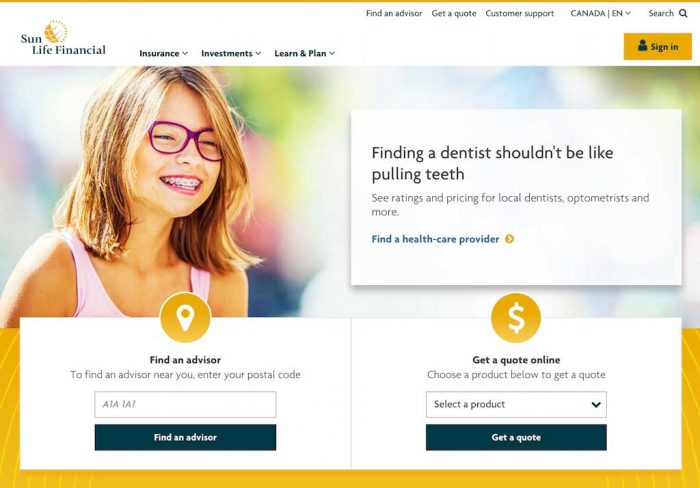Screenshot of the Sun Life Financial Website

At the top left of the screenshot, the Sun Life Financial logo is prominently displayed. The logo features a semi-circle: the left half is dark yellow, and the right half is white, adorned with yellow stripes radiating outward to provide a 3D, globe-like effect.

In the top right corner of the webpage, a series of navigation banners appear, including "Find an Advisor," "Get a Quote," and "Customer Support." Next to these is a language selection dropdown menu, currently displaying "Canada EN" for English. Further right, there is a search bar, and directly below it, a yellow "Sign In" button indicates that the user is not currently signed in.

Beneath the top banner, on the left side, a navigation menu offers additional tabs labeled "Insurance," "Investments," and "Learn and Plan."

The main content area features an image at the top left of a smiling woman with blonde hair, red glasses, and her eyes closed, showcasing her teeth in an exuberant smile. Directly to the right of this image is a text blurb that reads, "Finding a dentist shouldn’t be like pulling teeth. Find a health care provider, see ratings and pricing for local dentists, optometrists, and more."